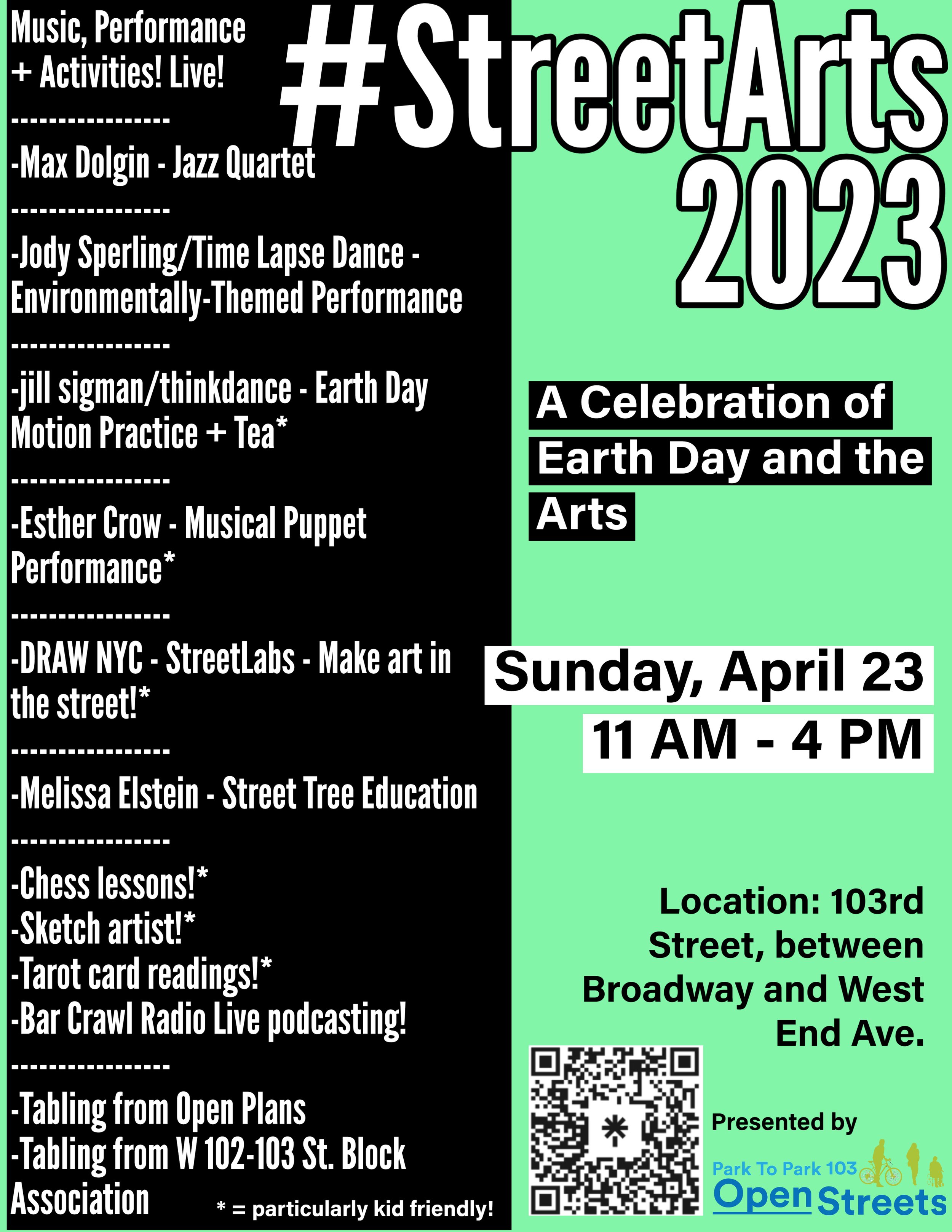This promotional flyer is divided vertically into two halves: the left side featuring a black background and the right side in light green. At the upper right corner, the flyer reads "Hashtag Street Arts 2023" followed by "A celebration of Earth Day in the Arts." Below this, the event details are listed: "Sunday, April 23rd, 11 AM to 4 PM, location: 103rd Street between Broadway and West End Ave." A QR code is also present with the note "Presented by Park to Park 103 Open Streets."

On the black side of the flyer, various activities and performances are detailed in white text:
- **Music, Performances, and Activities Live**:
  - Max Dolgan Jazz Quartet
  - Jody Spurling: Time Lapse Dance, an environmentally themed performance
  - Jill Sigman: Motion Practice and Tea
  - Esther Crow: Musical Puppet Performance
  - Draw NYC Street Labs: Make Art in the Street
  - Melissa Elstein: Street Tree Education
  - Chess Lessons
  - Sketch Artists
  - Tarot Card Readings
  - Bar Crawl Radio Live Podcasting
  - Tabling from Open Plans
  - Tabling from West 102 to 103 Street Block Association

Particularly kid-friendly activities are denoted with asterisks. The flyer also includes an outline of a person on a bicycle and another figure, possibly an adult and a child, illustrating the community and family-friendly nature of the event.